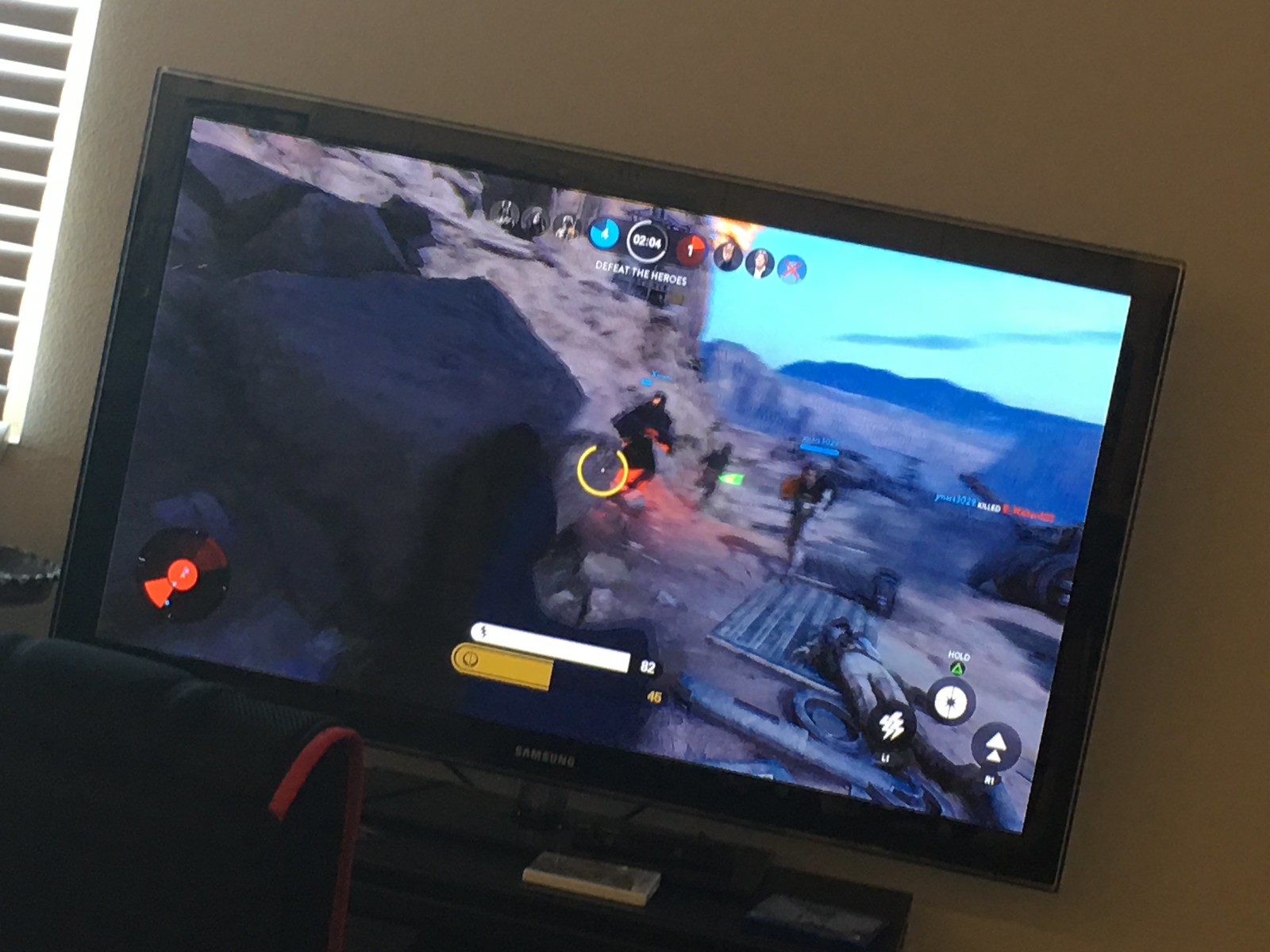A vivid, sideways snapshot captures a widescreen Samsung computer monitor displaying an action-packed video game. The digital scene teems with vibrant colors, showcasing an outdoor environment featuring dynamic elements like rocks, lasers, and characters both in motion and collapsed on the ground. The game's interface is visible, with the text “Defeat the Heroes” prominently displayed at the top, and various control icons lining the right-hand side of the screen. To the left, the edge of a gaming chair intrudes into the frame, while sunlight filters through window blinds, illuminating the scene from the upper left corner. The setup rests against a backdrop of soft, neutral tones, with a remote control conveniently placed on the table supporting the monitor.